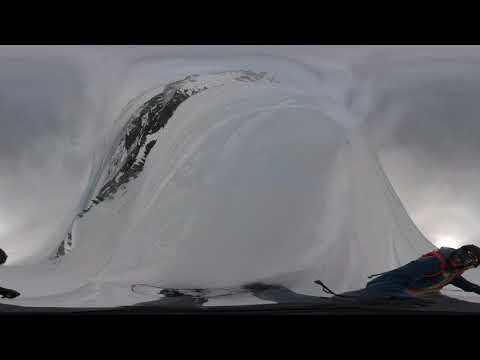The image showcases a skier navigating down a steep, nearly vertical ski slope. The skier, positioned in the lower right corner, leans forward with his head over his skis, wearing a dark blue jacket with straps suggesting he might be equipped with a parachute. His face is obscured by ski goggles, highlighting his intense focus. The mountain backdrop appears as a surreal, wave-like form rising majestically with a mix of snow-covered and tree-dotted areas. The sky overhead is wintry, filled with gray and white clouds. The photograph has a distinctive, abstract quality, achieved through the use of panoramic and barrel filters, and specialized lenses, creating a distorted yet compelling visual. Black horizontal strips frame the top and bottom of the image, adding to the artistic manipulation that accentuates the contrast between the monochromatic tones of the snow, skier, and sky.